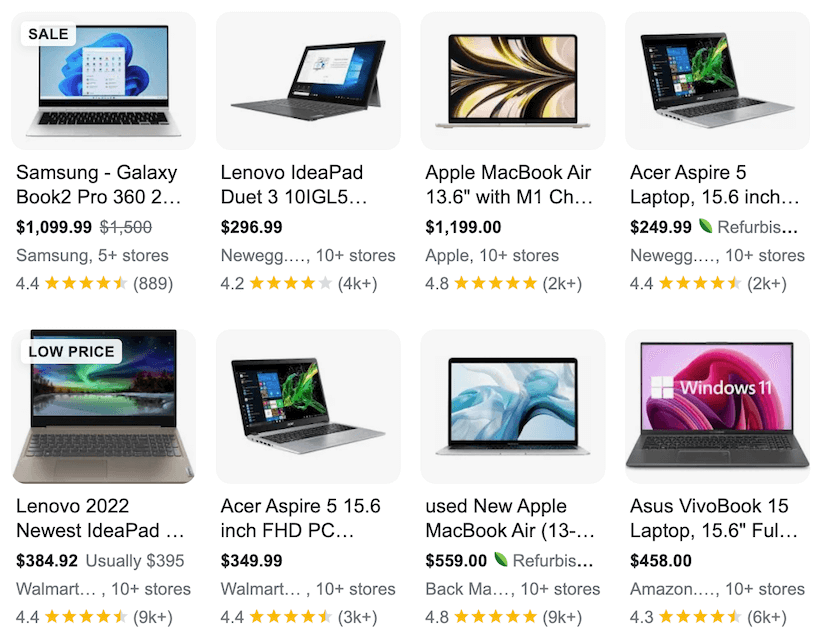This webpage showcases a selection of laptops arranged in two rows, each row containing four laptops. In the upper left corner of the page, the word "Sale" indicates that most of these laptops are offered at discounted prices.

**Top Row, from Left to Right:**
1. **Samsung Galaxy Book 2 Pro**: This laptop features a blue screen. Below the product name, details such as the price, brand, number of stores where it's available, and the user rating are listed.
2. **Lenovo IdeaPad Duet 3**: Displayed with the laptop itself facing slightly to the left, providing a clear view of its design.
3. **Apple MacBook Air, 13.6 inches with M1**: The screen displays a visually appealing design resembling mixed colors of paint dragged vertically with a toothpick.
4. **Acer Aspire 5, 15.6 inches**: This laptop, which is facing right, features a large green splatter design on its screen. A tag underneath states "Low Price," indicating a budget-friendly option.

**Bottom Row, from Left to Right:**
1. **Lenovo 2022 Newest IdeaPad**: Positioned forward, its screen showcases an impressive Aurora Borealis-like design set against a night sky.
2. **Acer Aspire 5, 15.6 inches FHD PC**: Similar to its counterpart in the top row, this model is facing right with the same green splatter design on the screen.
3. **Used/New Apple MacBook Air**: This laptop, facing forward, features an abstract blue and white design on its screen, suggesting a blend of modernity and minimalism.
4. **Asus VivoBook 15, 15.6 inches**: Also facing forward, its screen displays an abstract pink design with the "Windows 11" inscription spreading across the display.

Each laptop is carefully described with engaging details about its design and display, making it easier for shoppers to compare and choose the best fit for their needs.